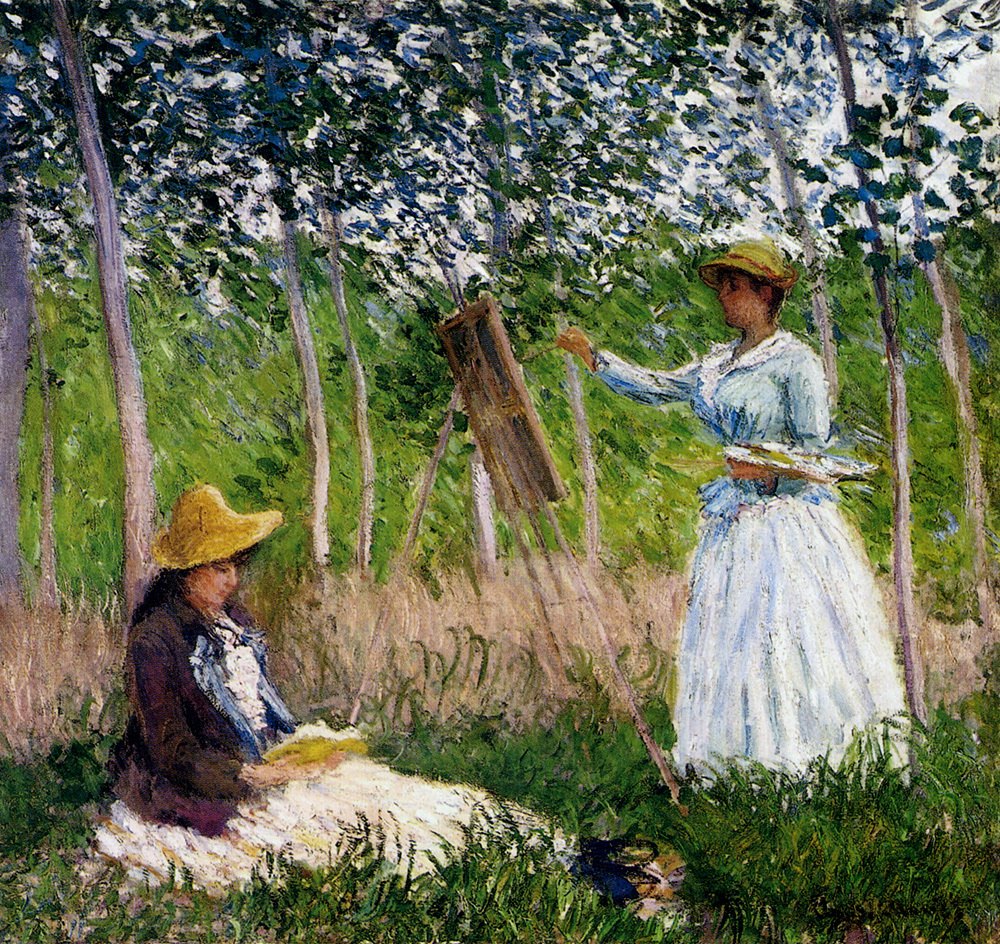This impressionistic painting, likely set in the 1800s, vividly depicts a serene outdoor scene featuring two women immersed in their activities amidst a backdrop of trees and long grass. The focal point is a woman standing and painting, dressed in a flowing light blue gown and a small yellow straw hat, delicately holding a palette in her left hand and a brush in her right, as she works at an easel. In the foreground, a woman in a light yellow dress and wide-brimmed straw hat sits on the ground, absorbed in a book. The surroundings are lush, with many green trees providing a verdant backdrop. The sky overhead is a muted light gray, adding a touch of melancholy to the tranquil setting. The color palette is primarily composed of pastel tones, with notable colors being green, light blue, yellow, and hints of purple. The painting beautifully captures a moment of calm and creative endeavor, rendered in an impressionistic style with fragmented brushstrokes that evoke a dreamy, almost otherworldly quality.